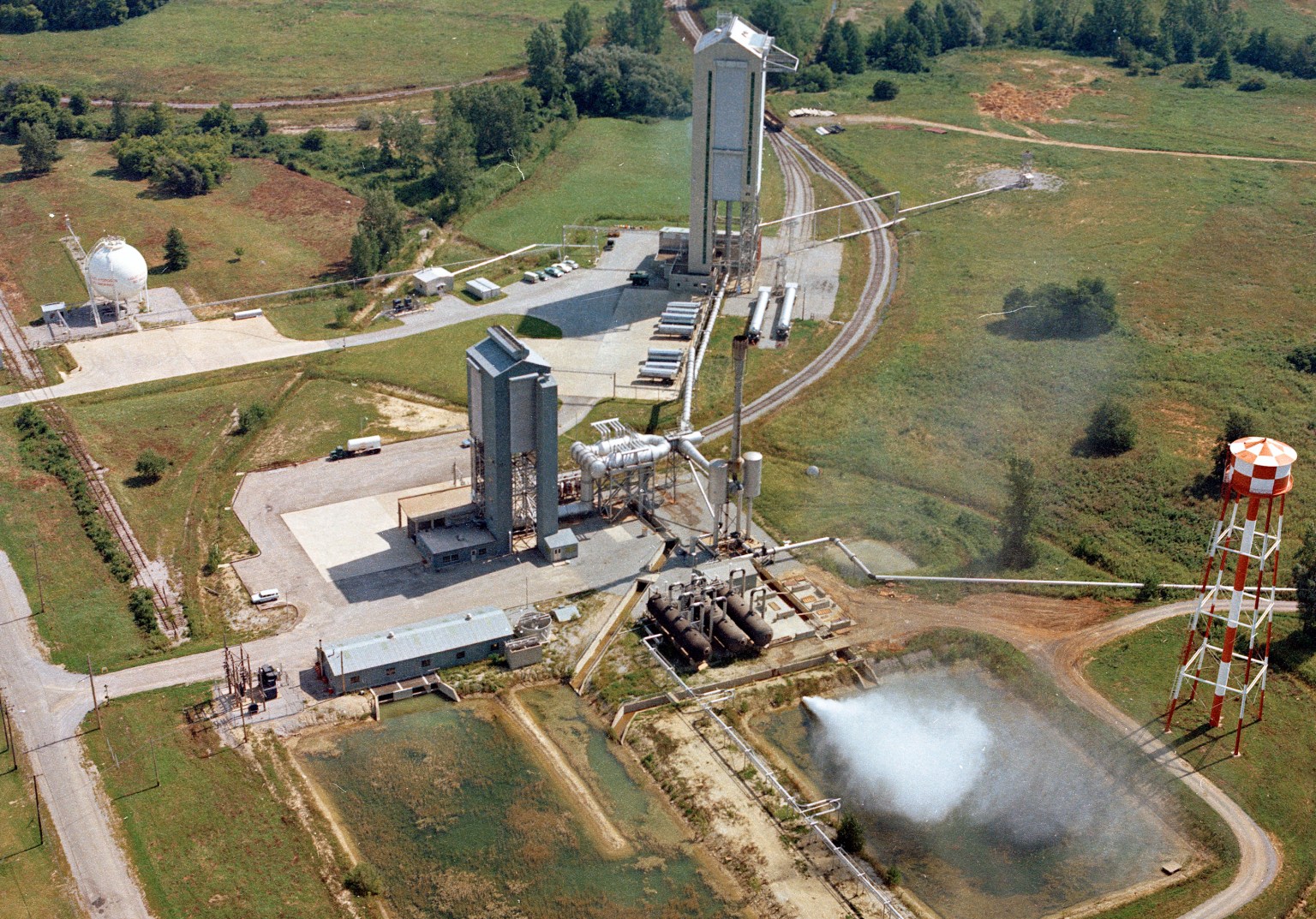This aerial photograph captures an extensive industrial facility situated on a lush grassy plain interspersed with trees. Prominent in the image, on the left, an asphalt road extends from the bottom left corner toward the center, leading into a large paved area dominated by two tall towers. The foremost tower, bluish and silver with numerous pipes, channels to the right towards black storage tanks, and downward to stagnant pools of water. The pipes further ascend from the first tower to connect with an even taller beige and white tower in the distant background. To the right of these pipes and pools, a red and white checkered water tower stands on a lattice structure. Curving train tracks arc from the middle top frame down and leftwards towards the blue and silver tower. Nearby, the top left of the frame features a spherical white tank adorned with red, though unreadable, text. Scattered trees form a backdrop to this industrial expanse. Additionally, various buildings are scattered around, including what appears to be watchtowers and several parked cars, suggesting active operations. There is a square pool with white spray near the red and white water tower, enhancing the scene's industrial complexity and adding to the dense network of infrastructure depicted in this vibrant yet industrious landscape.